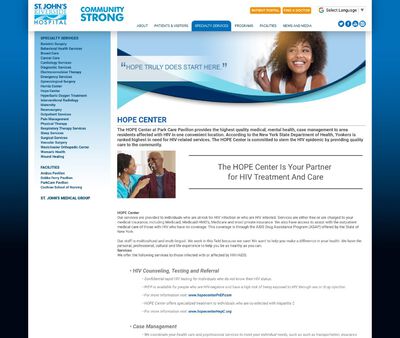The webpage for St. John's Riverside Hospital, focusing on the Community Strong initiative, prominently features the Hope Center as a partner for HIV treatment and care. The header banner showcases a smiling young black woman, accompanied by the uplifting quote, "Hope truly does start here." Below, another image displays a compassionate scene where a nurse provides comfort to an older black man, suggesting quality care and reassurance. The webpage offers various navigation links across the top and left side, though the text is notably small and hard to read. Social media links are conveniently located in the top right corner, and users have the option to change the language. Subtle vertical bars on the page's background transition from blue at the top to black as you scroll down, visually reinforcing the seriousness and support offered for individuals dealing with HIV.